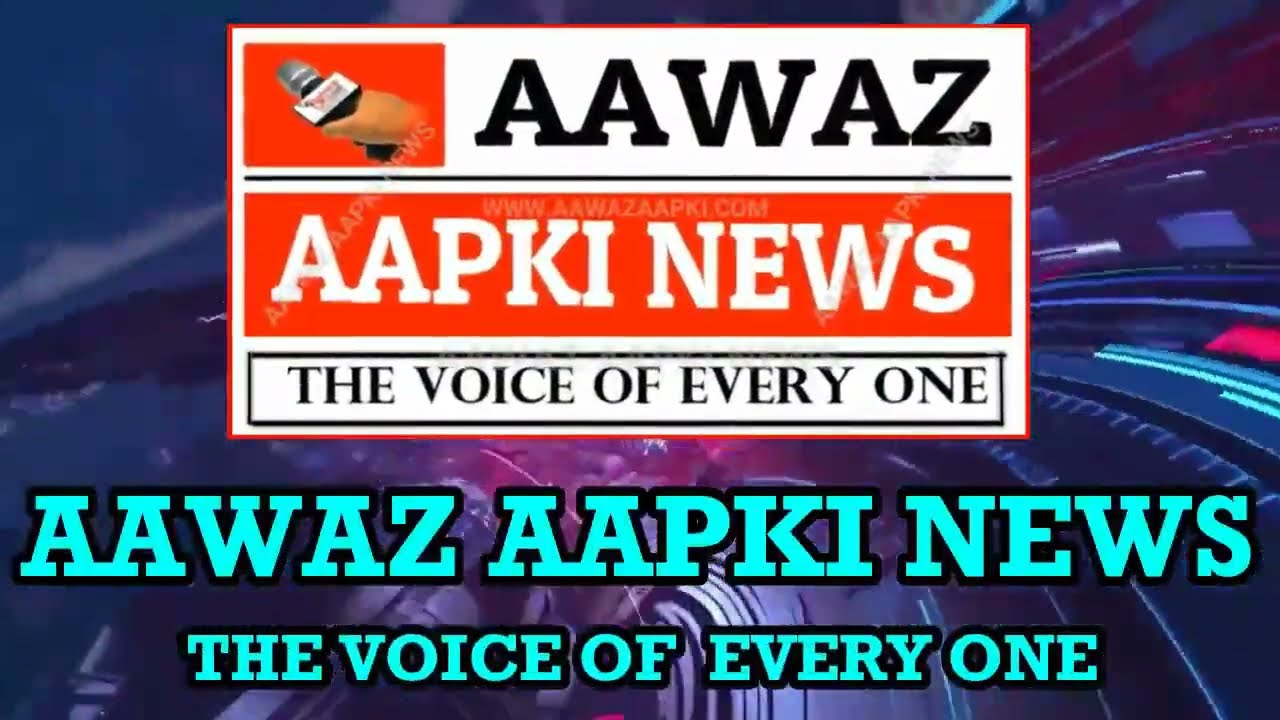The image appears to be a promotional graphic or screenshot from a website or advertisement for a news outlet called "A-A-W-A-Z A-A-P-K-I-NEWS: The Voice of Everyone." The central focus of the image features a hand holding a microphone to the left of the main text. The text includes "A-A-W-A-Z" at the top, followed by "A-A-P-K-I-NEWS" in white lettering on a red rectangular background, and below that, "The Voice of Everyone" in a smaller rectangle. The text is accented by swirling, abstract designs and geometric shapes in various shades of black, white, red, blue, green, pink, and purple. The background of the image features a combination of dark blues and purples, with additional details such as a repetition of the phrase "A-A-W-A-Z A-A-P-K-I-NEWS: The Voice of Everyone" in turquoise lettering interspersed throughout. The image has a dynamic and colorful layout, suggesting an engaging and modern visual style for the news outlet's branding.